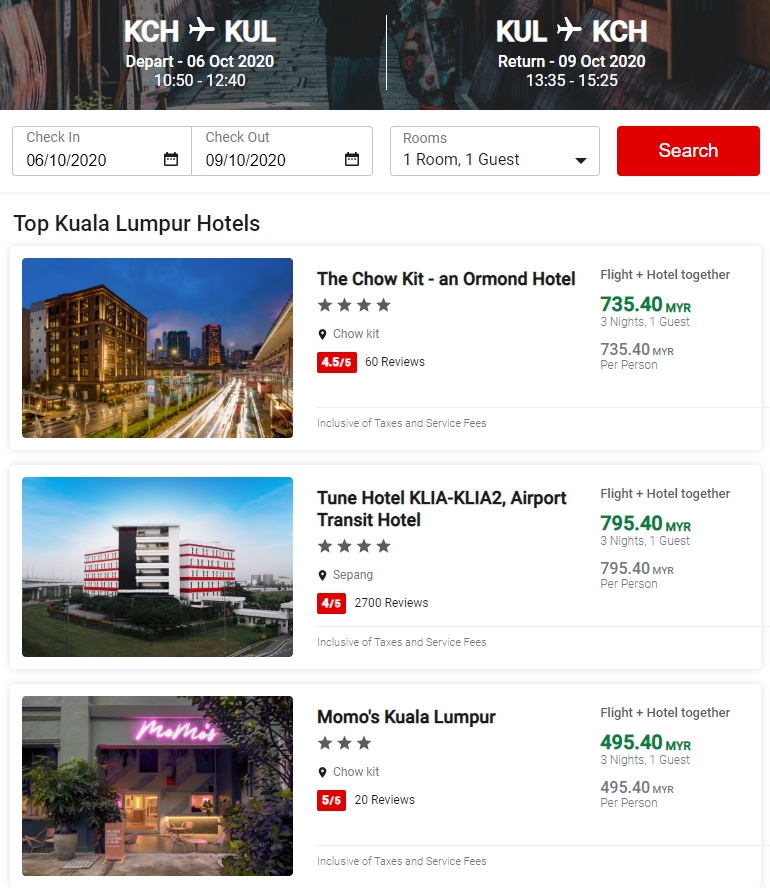**Web Page Overview: Top Kuala Lumpur Hotels Listing on KCHKUL**

This web page, presumably from the KCHKUL website, showcases listings for top hotels in Kuala Lumpur. The banner at the top of the page features a travel itinerary, with "KCH" followed by an airplane icon and "KUL" in uppercase letters. The departure date is listed as October 6, 2020, with a flight time from 10:50 to 12:40. The return trip is noted as October 9, 2020, from 13:35 to 15:25. Below this, the page offers check-in and check-out date options, displayed as "6/10/2020" and "9/10/2020" respectively. Room and guest selections are available via a dropdown menu, defaulting to one room for one guest, followed by a search bar.

At the center of the page, the heading "Top Kuala Lumpur Hotels" introduces three featured listings:

1. **Chow Kidd and Ormond Hotel**
   - Rating: 4 stars
   - Customer Reviews: 4.5 out of 5 based on 60 reviews

2. **Tune Hotel, KLIA-KLIA2 Airport Transport Hotel**
   - Rating: 4 stars
   - Customer Reviews: 4 out of 5 based on 2,700 reviews

3. **Momos Kuala Lumpur**
   - Rating: 5 stars
   - Customer Reviews: 5 out of 5 based on 20 reviews

This detailed display provides crucial information for travelers looking to book their stay in Kuala Lumpur, complete with ratings and a brief overview of customer feedback for each hotel.